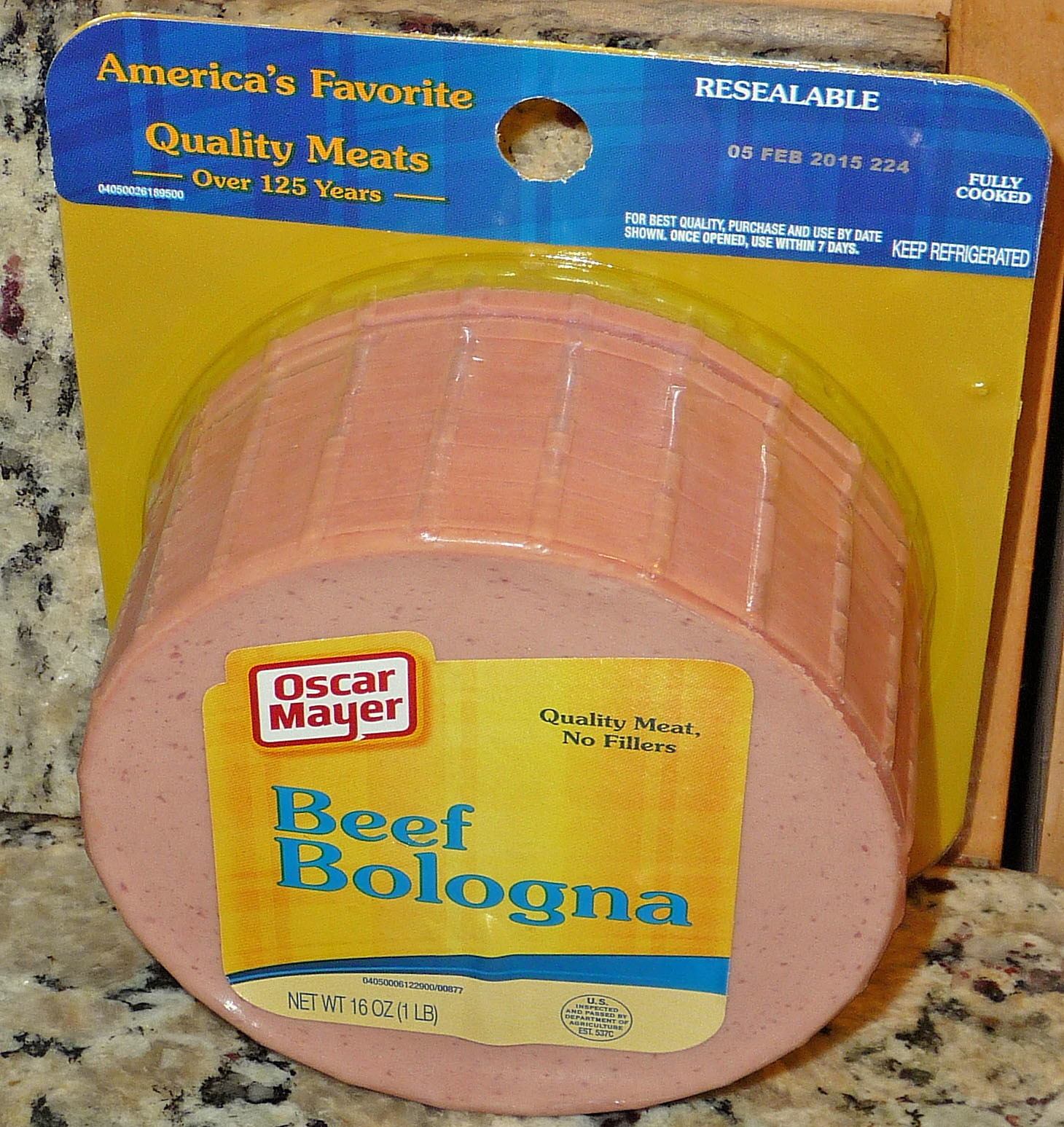This is an up-close image of Oscar Mayer's pre-sliced beef bologna in its packaging. The package features a prominent yellow and blue design with a bold red Oscar Mayer label. The top section of the package is emblazoned with gold lettering stating, "America's favorite quality meats, over 125 years." Additional text on the package includes "quality meat, no fillers," "resealable," and "fully cooked, keep refrigerated." The package includes a stamped expiration date of February 5, 2015. The bologna is stacked in a cylindrical form, tightly sealed in plastic. The package sits on a granite or marble countertop with a mottled off-white and black pattern, suggesting a kitchen setting.